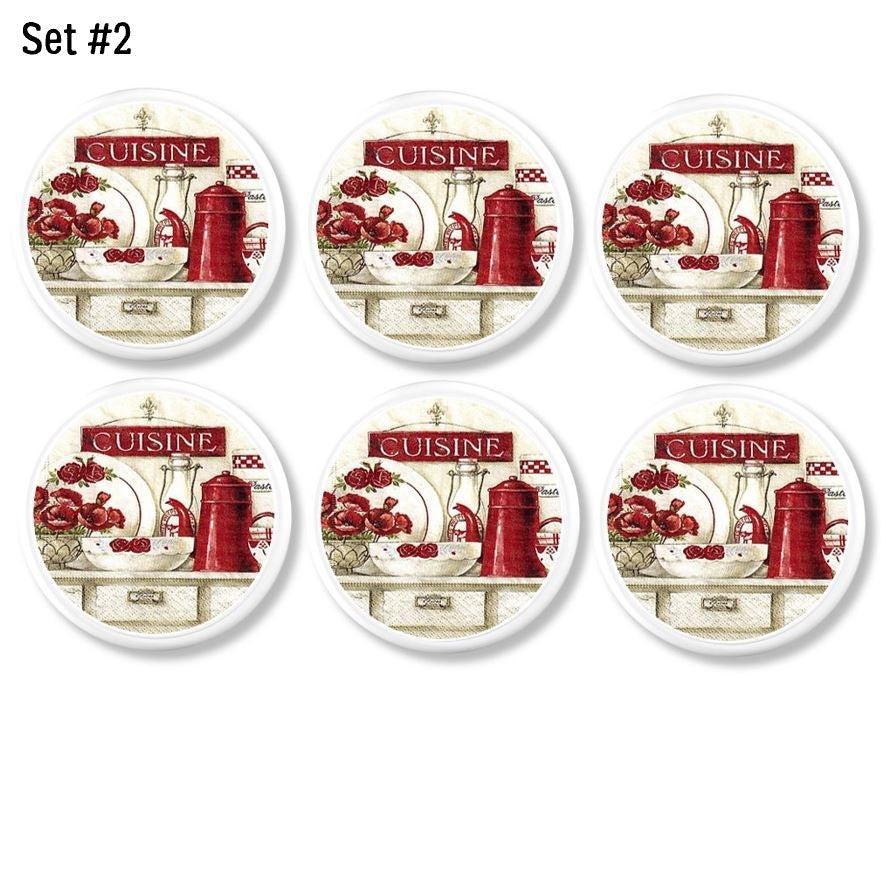The image titled "Set No. 2" depicts a set of six identical decorative plates or possibly coasters arranged in two rows of three. The plates are white ceramic with a country-themed illustration, characterized by red accents and a somewhat rustic style. Each plate features a prominent red sign reading "Cuisine," with a red teapot, resembling a hurricane lamp with a glass chimney, positioned to the right. To the left, there is a white plate adorned with red flowers, partially cut off in the illustration, and a white bowl with a red ribbon. The background includes a decorative plate with a floral pattern and what appears to be an oil lamp. The entire scene, set on a kitchen countertop above visible drawers, also includes a jar with a checkered red and white pattern near the top.